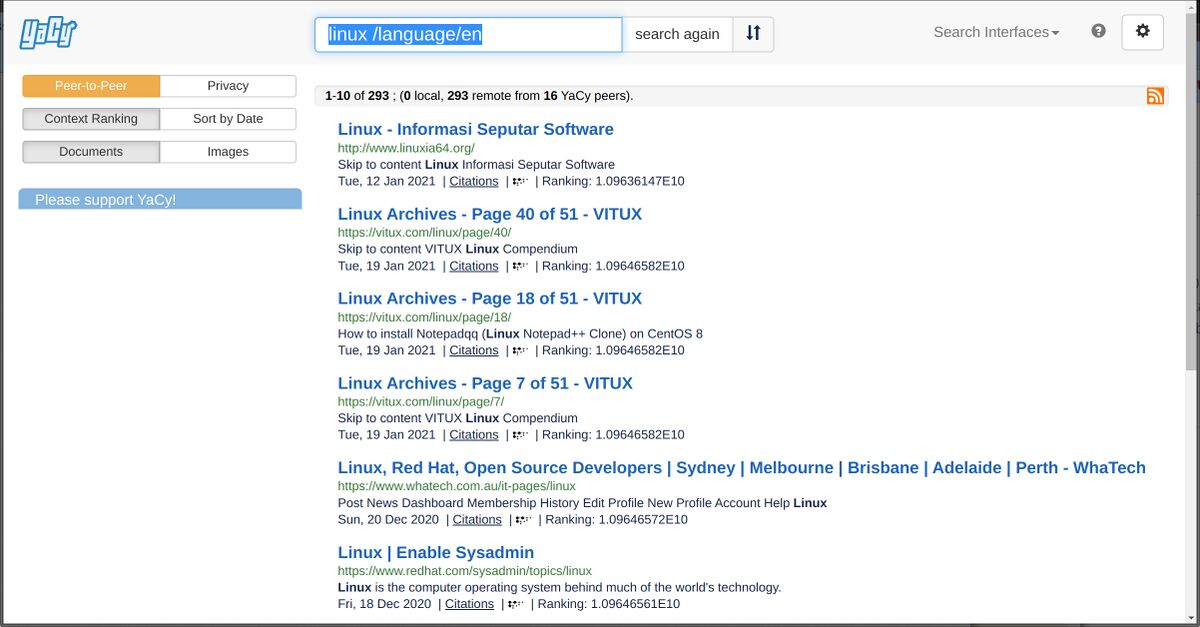The image depicts a webpage with a prominent banner at the top that reads "YACY" in bold letters. Below the banner, there are several clickable areas, each marked by distinct labels: an orange "Peer-to-Peer" button, a "Privacy" button, and another section labeled "Context Ranking." Additionally, there are options to sort search results by "Date," "Documents," and "Images." 

On the left side of the page, a button encourages users to "Please support YACY." The bulk of the page appears to be occupied by an extensive list of search results, many of which seem to pertain to Linux-related topics. Examples of these results include “Linux Inform YACY SEPTAR software,” “Linux Archives, page 40 of 51,” “Linux Archives, page 18 of 51,” and “Linux Archives, page 7 of 51.” Other entries mention “Linux Red Hat,” “Open Source Developers,” and “Linux/Enable System Admin,” with various dates noted beside them, such as 2020 and 2021. The page is densely packed with content, indicating a vast number of search results available for browsing.